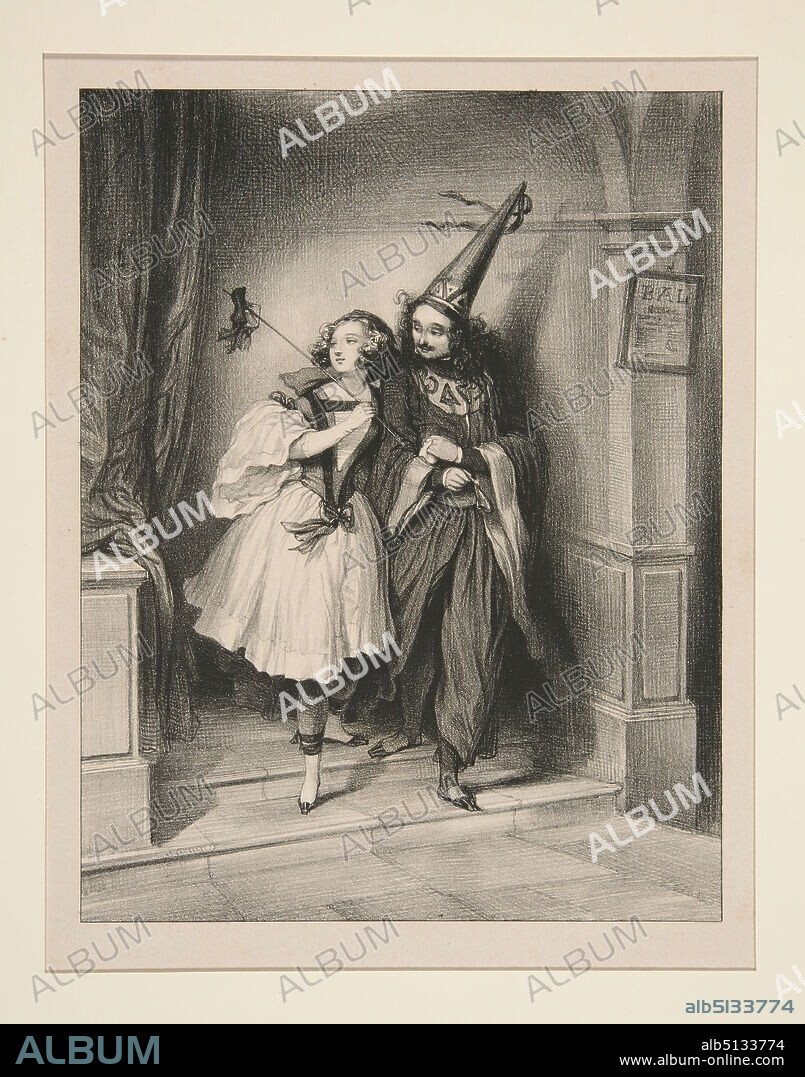This is a black and white scan or reproduction of an old illustration, potentially done in pencil or lead. The image features a young woman dressed in an old-fashioned white school dress with a bodice that ties at the bottom, holding a thin pole topped with a small horse figure. Walking arm-in-arm with her is a man adorned in elaborate wizard-like attire, including a tall conical hat with a tassel, a robe with a semi-circle collar and deep sleeves, a thin dark mustache, and long curly hair. They appear to be walking through an archway, possibly the entrance of a building or theater, with a sign on the right column that is illegible. The floor beneath them could be tile or wood, and a curtain is visible on the left side of the image. The illustration is surrounded by a double manila-colored frame. A diagonal watermark saying "ALBUM" repeats across the image, and at the bottom right corner, a black bar contains white text reading "ALB5133774" and "www.album-online.com". The watermark and the bar indicate that this is a purchasable reproduction likely available in an album from the aforementioned website.